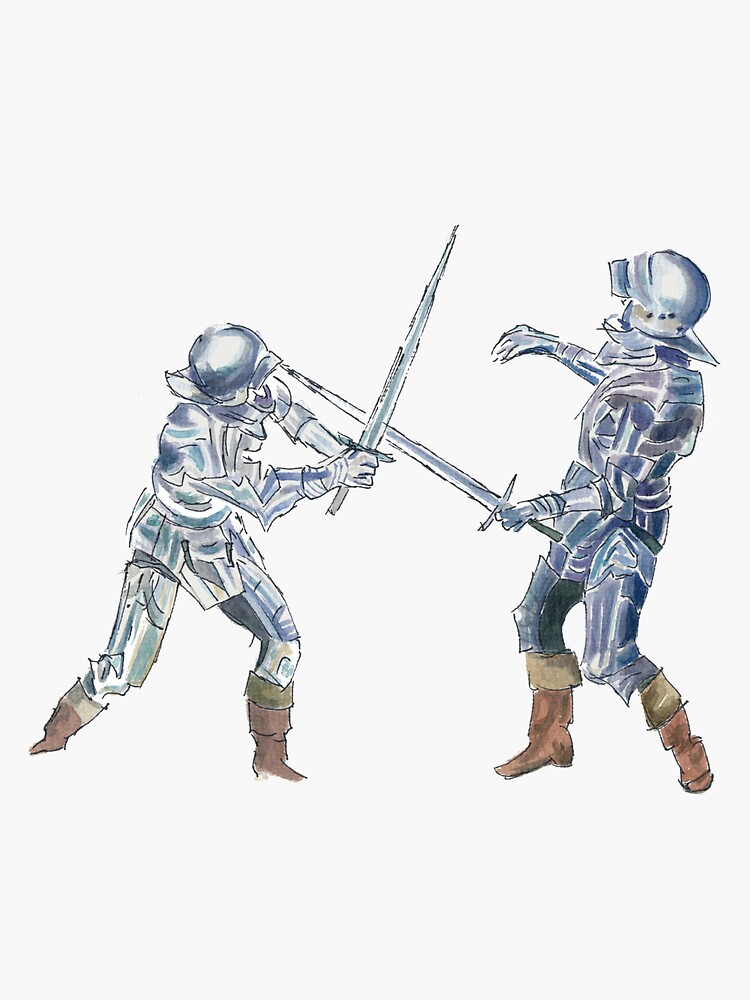This detailed drawing portrays an intense duel between two individuals, each clad in silver, metallic armor reminiscent of 16th to 18th century knights. Both characters are equipped with swords, poised mid-clash, and their posture suggests a tense and balanced standoff, with neither side appearing to win. They each wear distinctive boots, reaching just below the knees, featuring a lighter brown top rim and a darker brown body. Both combatants sport helmets as part of their matching silver armor, which has blue and green outlines adding subtle highlights. The background remains stark white, devoid of any additional elements or text, focusing all attention on the duel. The nature of the medium remains unspecified, it could range from watercolor to digital art. The piece lacks any identifying information about the artist or its setting, leaving its origins and placement a mystery.